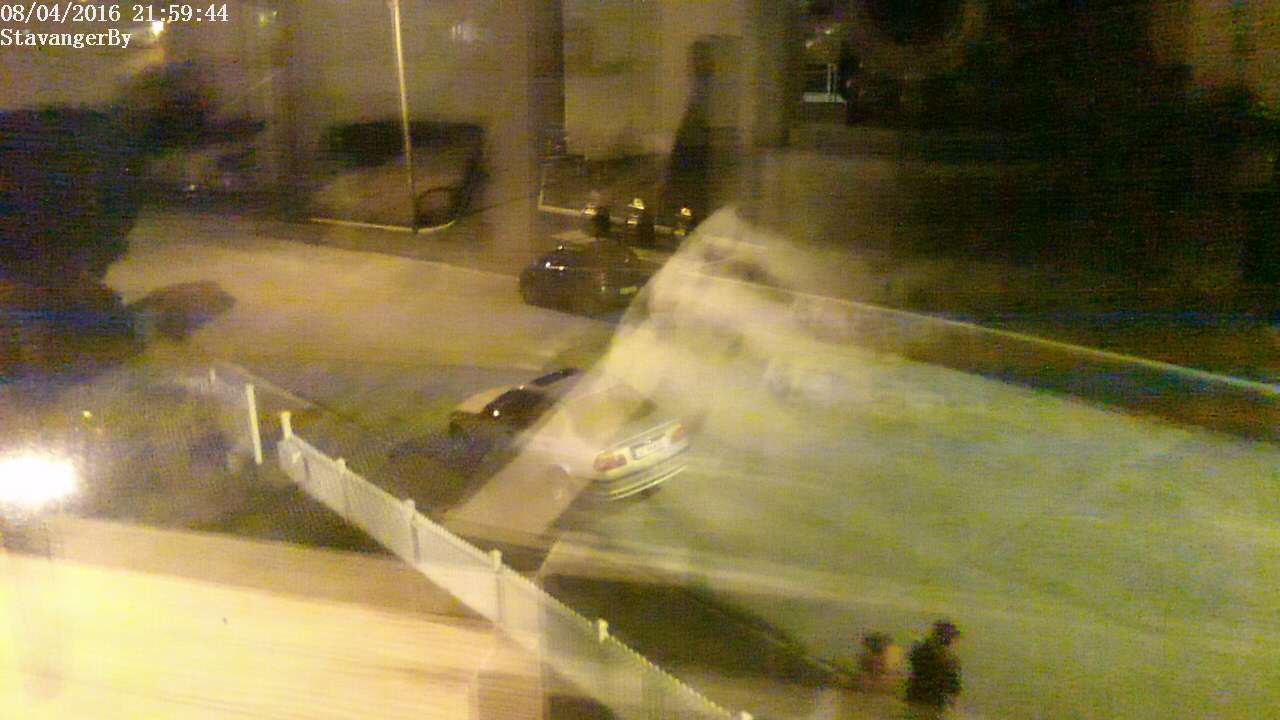This photograph, captured through a glass window, features the faint ghostly reflections typical of such images. Prominently towards the center and along the left edge, just before it crops out, a lens flare can be seen, indicating the flash's interaction with the glass. A timestamp on the upper left corner reads "08/04/2016 21:59:44." Below this, text displays "Stavanger By."

Outside the window, a street scene unfolds. A small silver car drives on a gray road, while another dark-colored car is parked at the roadside, adjacent to a short retaining wall. The background reveals large, blocky objects, possibly buildings, although the blur makes details indistinct. Two human figures, heavily blurred and partially cropped, are visible at the bottom of the image, adding to the overall sense of movement and liveliness in the scene.